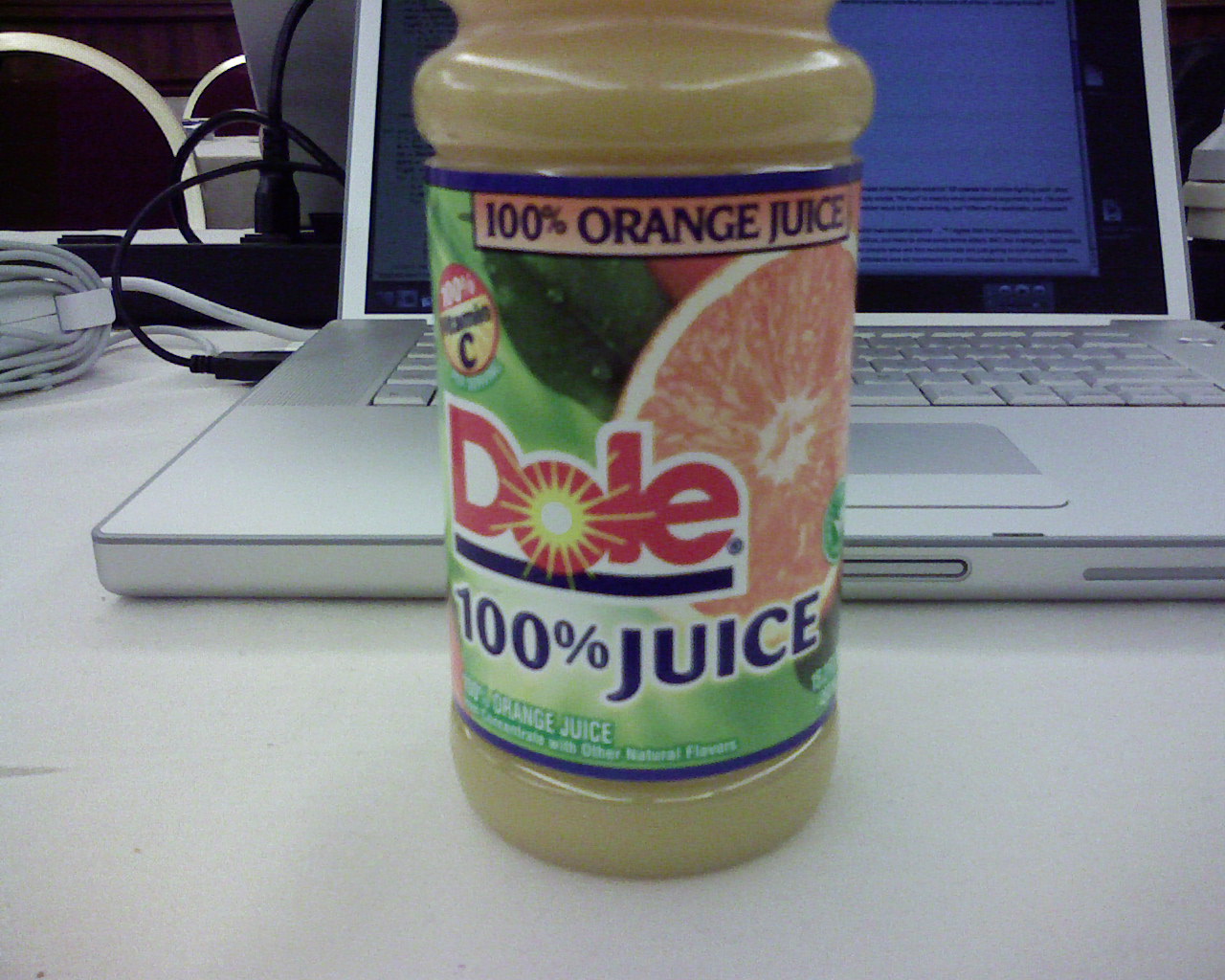The image is a close-up view of a clear plastic Dole orange juice bottle on what appears to be a white desk in an office or conference room setting. The bottle’s label is predominantly green, trimmed in blue, and prominently features a large orange sliced in half, displaying the fruit's pinkish-orange interior. The label includes the Dole logo with a yellow sunburst in the middle of the 'O', along with the text "100% orange juice" in blue letters at the top and "100% juice" below the logo. There is also a small circular label indicating "100% vitamin C". Behind the bottle sits a bulky, older-model silver laptop, which is turned on and appears to have a word processor open on the screen. Extension cords and a power strip are visible to the left, suggesting a workspace with multiple devices connected.